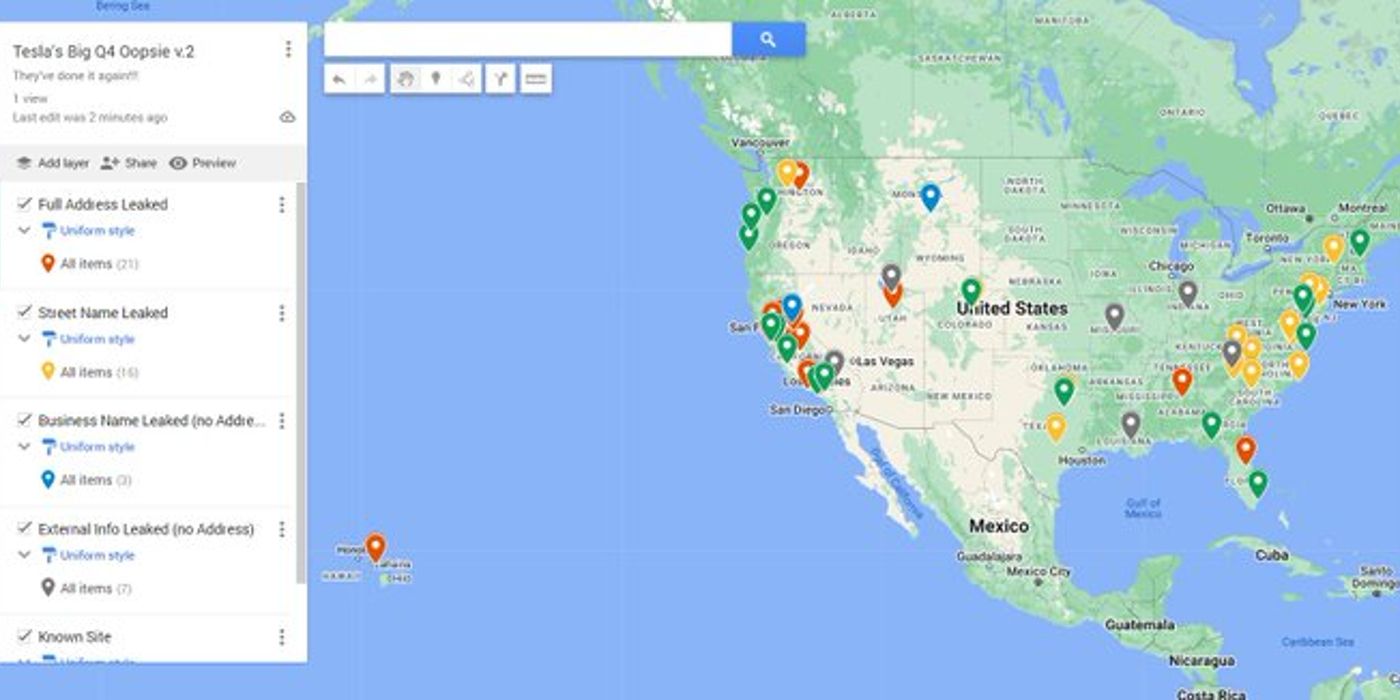In this image, we observe a detailed map screen of North America. On the left side, there is a white vertical column containing various options. At the top of this column, it reads, "Tesla’s Big Q4 V2." Below this header are five distinct categories, each sectioned with a white background. The map prominently features a large portion of the Pacific Ocean on the left, rendered in blue.

At the very top of the screen is a search bar accompanied by a blue search button. Directly below the search bar are four small white shapes, each containing different logos. Toward the right of the column, the map displays a significant portion of North America, including the United States, part of Canada, Greenland, Mexico, and Central American countries such as Guatemala and Costa Rica. The map also depicts Cuba and sections of the Atlantic Ocean and the Gulf of Mexico, both colored in blue.

The map is adorned with various colored icons: green, dark orange, light yellow, blue, and gray. These icons are distributed across the map, forming clusters on the west coast, the Midwest, and the east coast of the United States. The west coast in particular has a concentration of white, representing areas of interest. The image overall is a comprehensive visual representation of North America with specific emphasis on geographical and categorical data points.